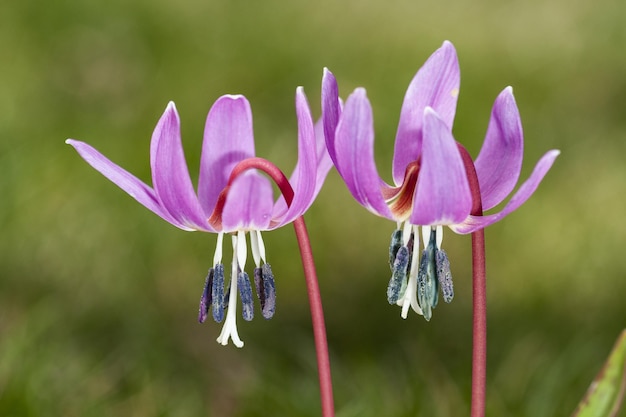This color photograph captures a close-up of two flowers, side by side, situated prominently against a backdrop of blurred green grass or garden foliage, creating a bokeh effect. The main subjects of the image are the flowers, each emerging from a delicately curved, light red stem resembling the shape of a candy cane. Both flowers stand at the same height with their vibrant purple petals gracefully facing upwards towards the sky. In contrast, the center parts of the flowers, containing the stamen and pistils, hang downwards. These downward-facing features have a light green base capped with distinctive purple or blue tips. The two flowers are closely aligned, so much so that a couple of their petals in the back overlap slightly. This intricate and detailed composition brings a fine balance between the vivid colors and the intricate shapes of the flowers, drawing the viewer's attention to their unique beauty.